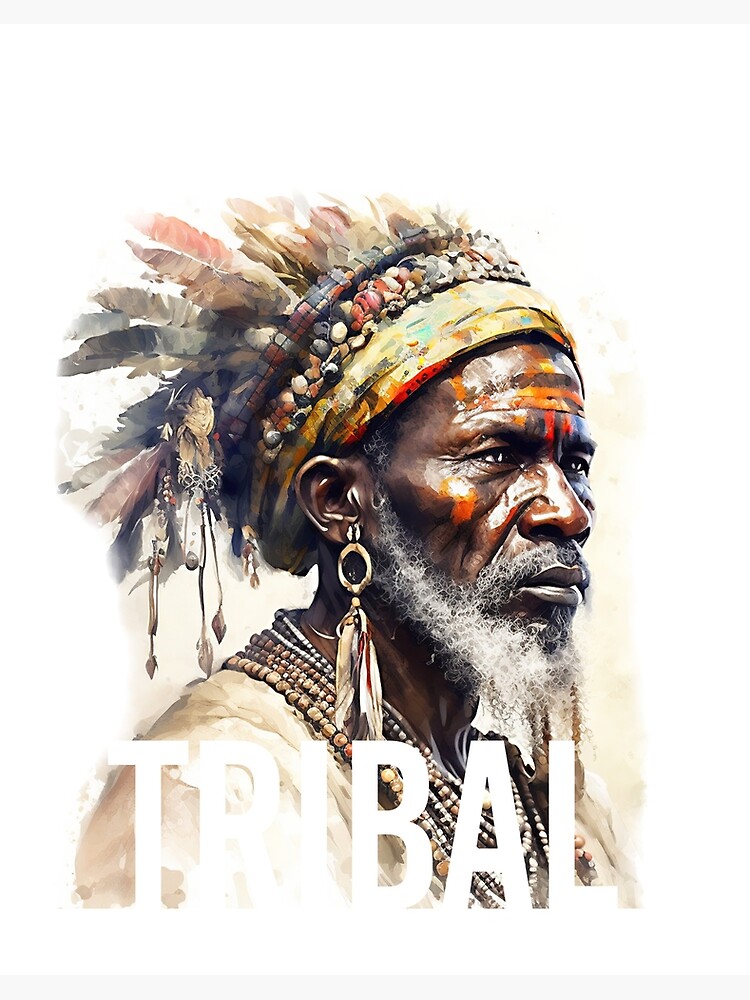The image depicts an older Black man with a dark complexion, a gray beard, and a black and white mustache. His face is slightly squinted, and he looks to the right with a serious expression. Notably, his face features ceremonial face paint in vibrant yellow, orange, and red hues, dripping down just above his eyebrows and accentuating his cheekbones. He wears a distinctive headband adorned with a yellow top stripe and a row of rock beads, which is further embellished with a cluster of purple and gray flowers pointing backward. Dangling from his ears are circular earrings, each with hanging feathers. Around his neck, he sports multiple beaded necklaces, adding to his elaborate attire. He is dressed in a detailed light gray shirt. Across the bottom of the image, the word “TRIBAL” is prominently displayed in all capital white letters. The background of the image is entirely white, highlighting the detailed traditional and tribal elements of his appearance.